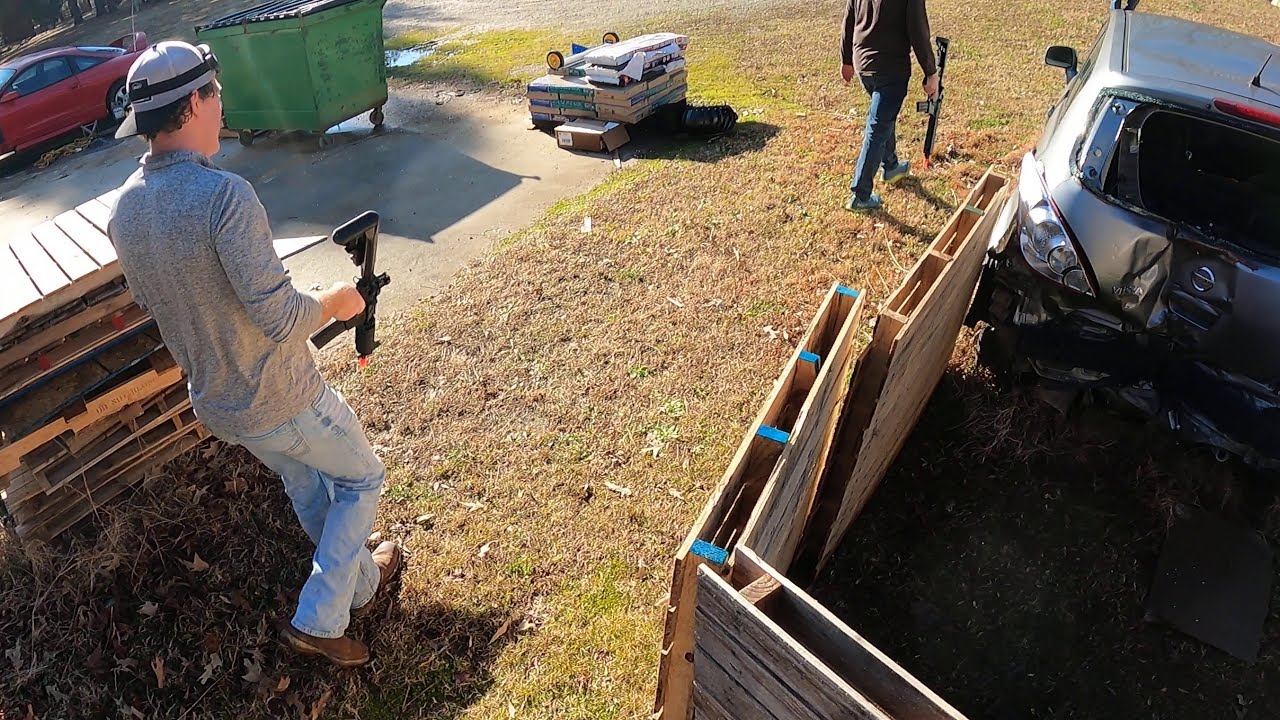The photograph captures an outdoor scene featuring two men walking through a field with patches of dead grass and fallen leaves. The image is taken from an elevated, sideways angle, allowing a view of various elements scattered around the area. On the right side, there's a silver car with a significantly dented front end, suggesting it has been in a crash. Leaned against the car are stacks of wooden pallets and crates, some of which appear to have dirt inside. To the left of the car is a man dressed in a gray, long-sleeved shirt with the sleeves pushed up, light blue jeans, brown shoes, and a gray hat. He is holding what appears to be a paintball gun or similar type of weapon. In front of him, another man, visible only from the back, wears a dark shirt, darker blue jeans, and blue shoes. He too carries a paintball gun. The left of the frame features more wooden pallets, random boxes, a green dumpster on wheels, and a parked red car. The atmosphere suggests an environment either for a game like paintball or a staged setting with the scattered items adding to the rugged, utilitarian feel of the location.